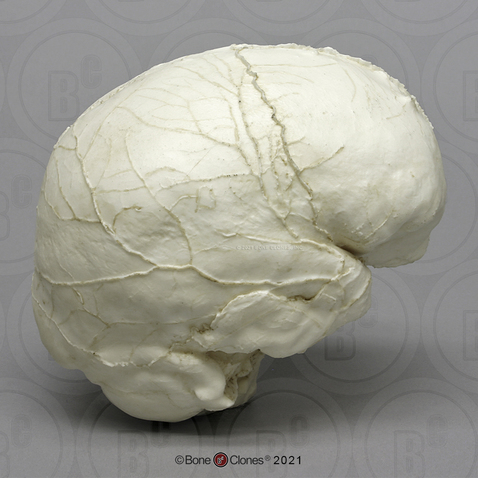This photograph features a detailed and smooth white replica of a human brain made from bone, complete with intricate vein-like structures that mimic the real brain's vascular details. The brain, which lacks the typical ridges, is propped up rather than lying flat, emphasizing its textured, vein-marked surface. The backdrop is a grey field adorned with multiple circles featuring a transparent "B" with a dark "C" positioned slightly above and to the right, resembling an exponent. Along the bottom of the image, the text "Bone Clones 2021" is prominently displayed, confirming the replica's creation date and manufacturer.